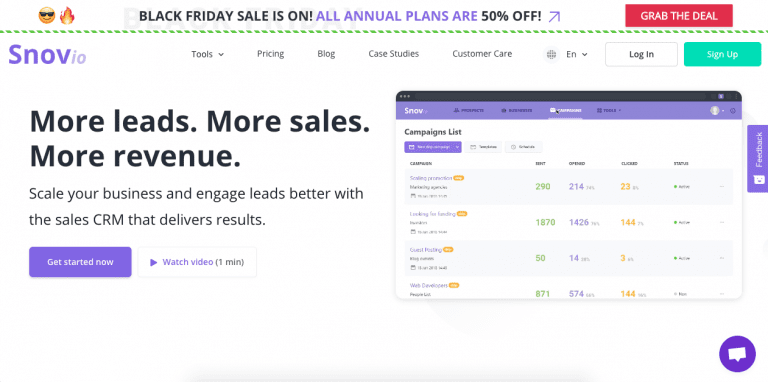Title: Black Friday Sale Advertisement Screenshot

Description: The image is a promotional banner advertising a Black Friday sale, featuring a lively and engaging design. At the very top, there is a playful smiley face icon wearing sunglasses alongside a fire emoji, enhancing the excitement of the sale. The bold text announces, "Black Friday Sale is On!" followed by a statement in purple that reads, "All Annual Plans are 50% Off." Below this text, an arrow points towards a prominent red button labeled "Grab the Deal."

On the upper section of the page, we see the brand name "SNOVO" prominently displayed, along with a navigational menu that includes links to "Tools," "Pricing," "Blog," "Case Studies," and "Customer Care," with an option to change the website's language to English or other available languages. Additionally, there are buttons for "Login" and a green "Sign Up" button.

A vibrant banner next to the main advertisement states, "More Leads, More Sales, More Revenue. Scale your business and engage leads better with the sales CRM that delivers results." It’s followed by a strong call to action with the text, "Get started now!" and a "Watch Video (1 minute)" button.

In the lower section of the screenshot, there is an embedded text box featuring an image of a campaign list, showcasing numbers and percentages that visually depict the campaign's success, reinforcing the effectiveness of the sales CRM being advertised.